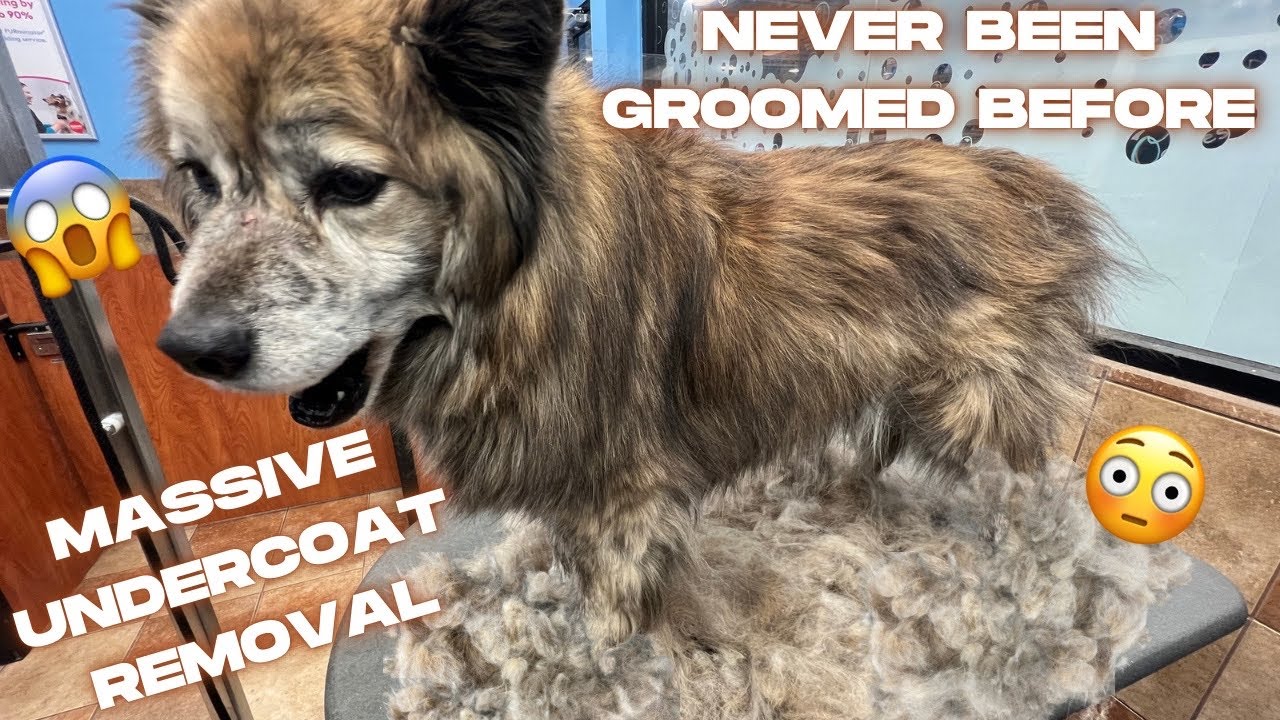The image is a horizontally oriented photograph depicting a small, brown dog with shades of light brown and dark brown, as well as a gray patch on its nose and around its eyes, standing amidst a massive pile of removed fur on a grooming table. The dog, appearing visibly unhappy, has black ears, a black nose, and black eyes, with the bottom part of its face showing some white fur. The background reveals a grooming room with blue walls, calendars, a white screen with pictures, wooden cabinets, and brown tile flooring. Captioned in white letters at the top, the text reads "Never been groomed before," while the lower left corner displays "Massive undercoat removal." Additionally, there are two yellow emoticons near the dog's face—one looking shocked and surprised, and the other looking sad.